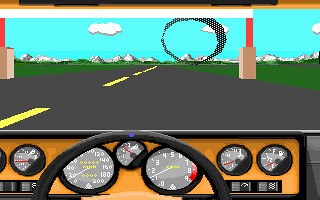In this rectangular image, we are presented with a scene that resembles a still from a video game, depicted from a first-person perspective as though the viewer is seated behind a steering wheel. The steering wheel is centrally positioned, emerging from the bottom edge of the image. Directly ahead, a light amber-colored dashboard houses various circular dials and gauges. These instruments appear to measure metrics such as speed (in MPHs), RPMs, and possibly a clock, although the specifics are somewhat unclear. To the right of the dashboard, there is a visible fuel gauge indicating a quarter tank of gas remaining. The road ahead is dark and paved, flanked on either side by vibrant green grass. The scene extends towards the horizon where majestic, white-capped mountains meet a clear, blue sky, creating a picturesque backdrop for this virtual driving experience.